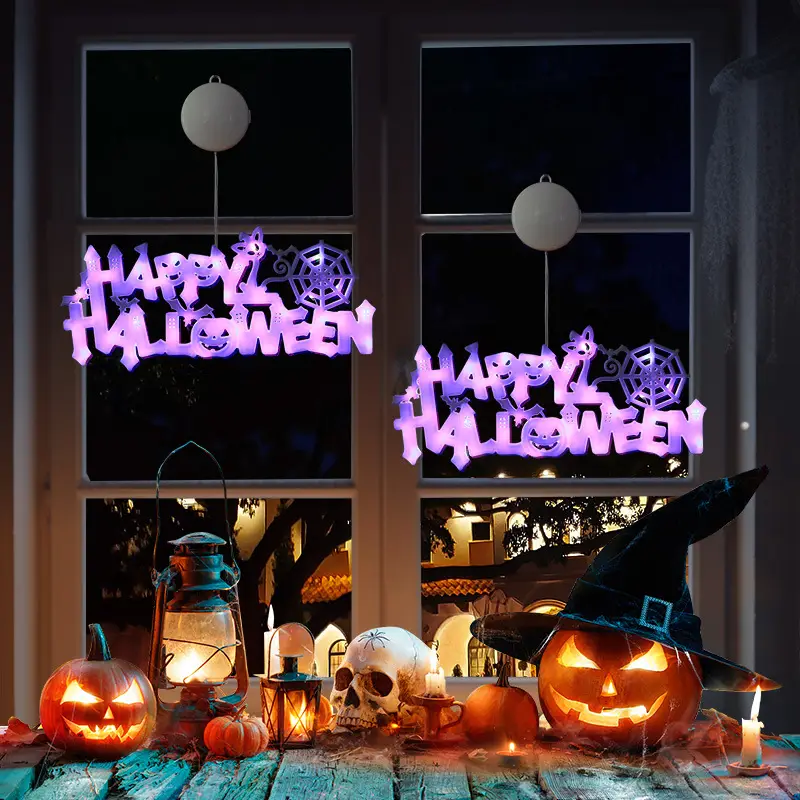This detailed Halloween-themed photograph showcases a collection of festive decorations arranged in front of what appears to be a window. The scene features two carved jack-o'-lanterns on either corner of the frame, their eerie faces illuminated by candles placed inside them. The pumpkin on the right is adorned with a black witch's hat, adding an extra spooky touch. Centered at the bottom is a human skull, which has a spider design drawn on its forehead. Surrounding the skull are several lit candles and mini pumpkins resting on the wooden deck. To its left, a large lantern with a candle inside casts a warm glow on the tableau.

Hanging from the window are two bright purple LED signs that read "Happy Halloween," each accompanied by decorative elements like spiderwebs, cats, and pumpkins. Through the glass, there is a reflection of a neighboring, well-lit Spanish Mediterranean-style house, suggesting that it is nighttime. The overall composition of this image, including the various lights and decorations, creates a festive and spooky Halloween ambiance.